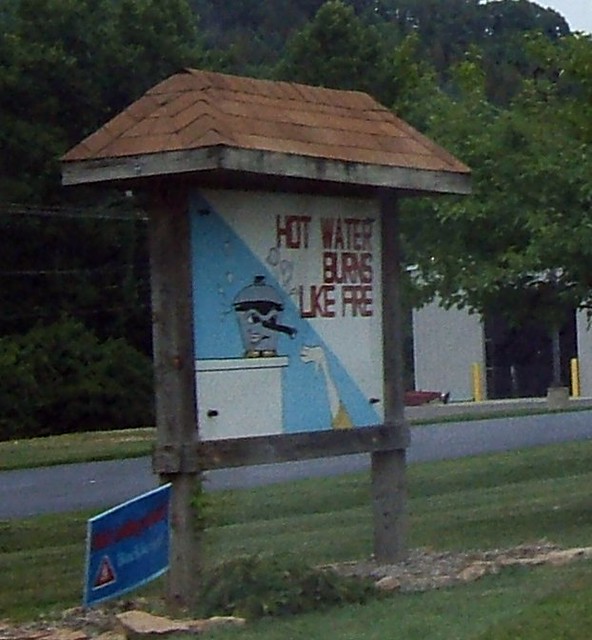The photograph appears to be taken through a glass window, possibly from a car or a house. The image prominently features a park sign in a verdant outdoor setting. Surrounding the sign are numerous trees, lush with green foliage, creating a serene, natural backdrop. To the right side of the image, partially obscured by trees, there is a white structure that seems to be a shed. Directly in front of the shed and trees, a patch of well-manicured grass transitions into a black asphalt road.

The park sign itself is positioned on the grassy area across the road. It is a sizable and eye-catching sign, complete with a decorative brick roof resembling a small shelter or awning. The sign carries an important safety message, reading, "Hot water burns like fire." The design features a mischievous-looking pot of water with a face, and a hand reaching up towards it, presumably a warning about the dangers of scalding hot water. The background of the sign is a combination of white and light blue hues.

Adjacent to this large sign, to the left, there is a smaller yard sign. This sign is primarily blue with red and white lettering, though the text is harder to discern due to the blurriness from the glass. It appears to convey a "buckle-up" safety message, urging viewers to use seat belts.

Overall, the scene captures a blend of natural beauty and public safety messaging, emphasizing precaution in a tranquil park setting.